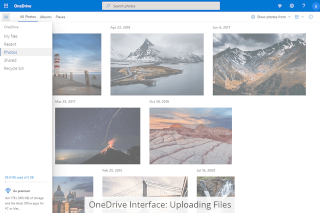A small, rectangular image depicting a screenshot of the OneDrive interface. At the top, there is a blue bar with a white Windows icon in the upper left corner, and "OneDrive" written to the right of it. The middle section features a white search box with indiscernible text, accompanied by four small, white icons to the right. Below this, a white area displays three menu options in black text on the left side, with the leftmost one highlighted by a blue bar, although the text is too small to read. Additional text and icons are visible in the upper right corner, but also too small to discern. 

On the far left, a rectangular panel contains five clickable options, the third one highlighted in gray. Towards the bottom of this panel, more blue text is present, but again too small to decipher. Adjacent to this is a white box with a blue icon and black text to the right, followed by additional black text below.

The image is primarily dominated by two full pictures and four partial pictures. The upper center image shows an Arctic mountain scene with an overcast sky and snow, accompanied by indiscernible text, possibly dates, above them. To the left is half of a picture featuring a lighthouse against a blue sky, while the rightmost image on this row displays a snow-covered mountain. Below these, a partial image depicts a nighttime volcano with flowing lava, adjacent to an image of salt flats at sunset. 

The bottom row contains three smaller, harder-to-see images: the leftmost possibly shows a cathedral or domed building at dusk; the middle image is unclear, though it might depict part of a suspension bridge; and the rightmost image is ambiguous, possibly showing part of a waterfall. Overlapping these bottom pictures is a white box with black text that reads, "OneDrive interface uploading files." This heavily implies the screenshot is from a OneDrive interface displaying various uploaded pictures.